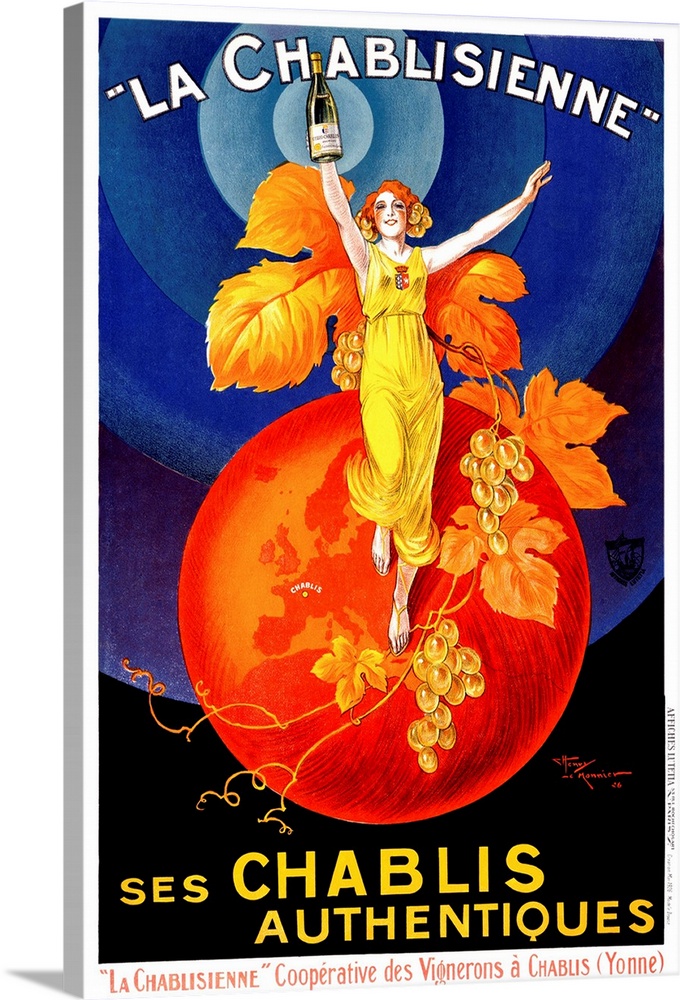This is a photograph of a vintage-style Art Deco advertisement for Chablis wine. The book cover features white text at the top that reads "La Chablisienne," slightly curved around the edge. At the center of the cover is an illustration of a cheerful orange-haired woman with golden curls, made to look as though her hair is crafted from grapes. She is holding up a bottle of white wine with a joyful expression. The woman is depicted wearing a flowing white dress adorned with a shield on her chest, colored blue on the left and red on the right, and sandals with dangling straps.

Behind her, an orange globe prominently displaying Europe and a small dot labeled "Chablis," indicates the wine's French origin. The globe is adorned with orange leaves extending down into vines with golden grapes. The rich warm tones of the woman and globe contrast against the dark blue background. Below the illustration, in bold yellow text, the words "Chablis Authentiques" highlight the authenticity of the Chablis wine. At the very bottom, a smaller text includes "La Chablisienne Cooperativa de la Vignerons Chablis (Yonne)," indicating the cooperative group responsible for the wine.